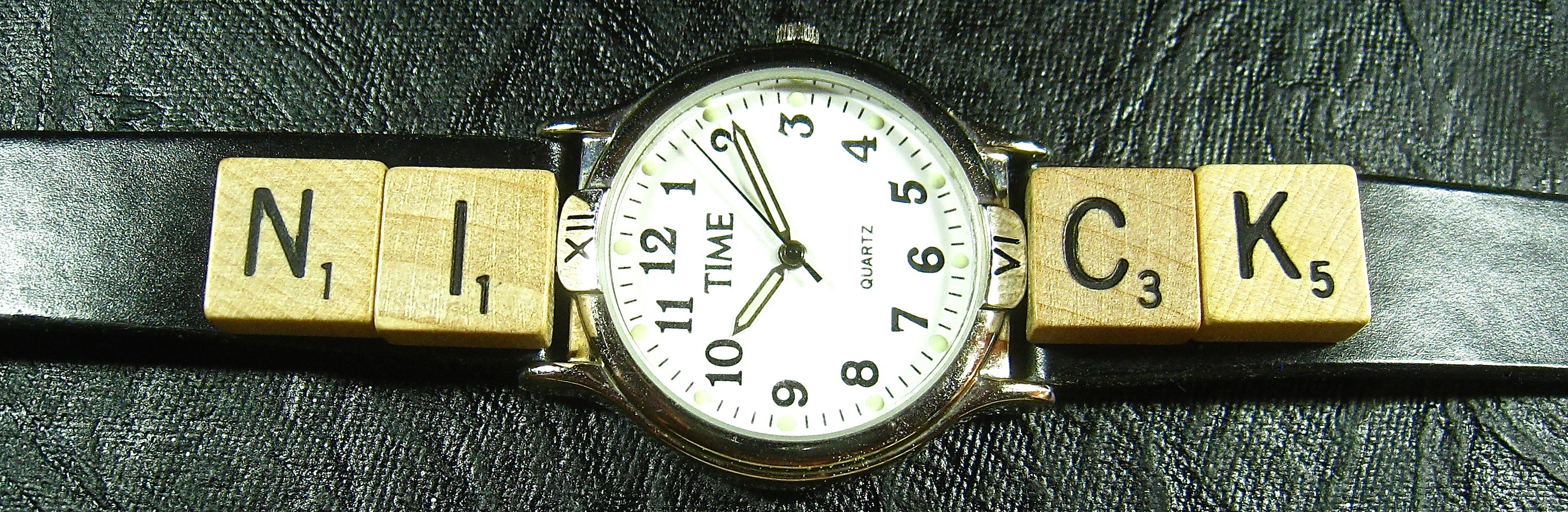A detailed caption for the image could be:

"In a rectangular image centered on a wristwatch, the watch lies horizontally against a plush leather background. With a polished silver case and a sophisticated white dial, the timepiece features black numerals in a classic format—eschewing Roman numerals for traditional digits. The word 'TIME' is elegantly inscribed at the top of the dial, while 'QUARTZ' is prominently displayed at the bottom. The wristwatch is complemented by a sleek black leather band. Adding a playful twist, Scrabble tiles are artfully arranged above the band: 'NI' to the left of the watch face and 'CK' to the right, playfully forming the word 'NICK' when read from left to right."